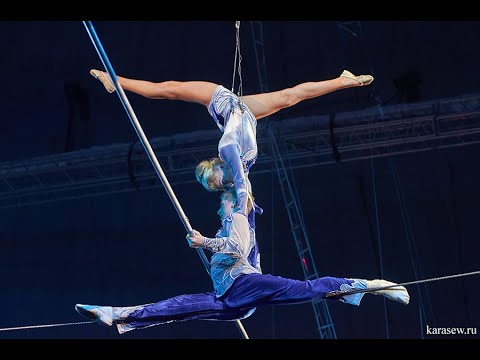This photograph captures an impressive indoor performance by two circus acrobats dressed in light blue and gray outfits. Central to the image is a man performing a split on a high wire, his legs fully extended with one foot pointing to the left and the other to the right. He maintains his balance using a long metal pole that he grips with both hands, holding it perpendicular to the wire. He is barefoot, and his blue costume includes long pants.

Balancing atop him is a woman with blonde hair styled in a bun. She mirrors his split-legged position, creating a symmetrical visual effect. Her legs are stretched outward as far as possible, adorned with gold slippers. She supports herself by placing her hands on the man's shoulders, her face just above his head, forming an elegant pose. The background is dark, accentuating the performers against the dimly-lit setting, and other indistinct figures can be seen, adding depth to the scene.